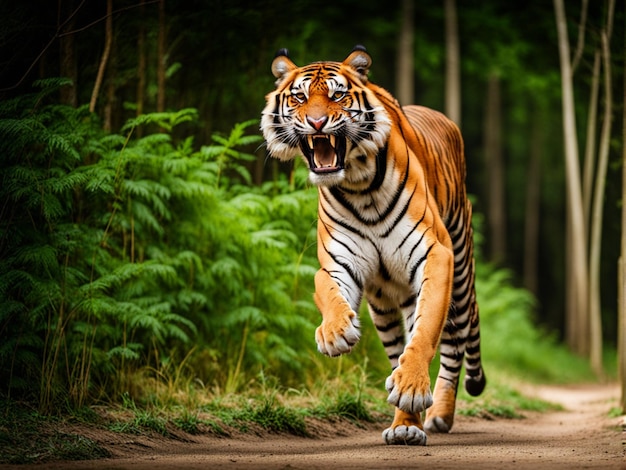This is an up-close, dynamic photograph of a roaring tiger running directly toward the camera, mid-stride with its front paws lifted off the ground. The tiger's mouth is wide open, showcasing its sharp upper and lower canines and a pink tongue that transitions to a darker shade. Its fur is a striking mix of orange and black stripes with a white underside, which extends to its legs and under its jaws, highlighting its powerful physique. The tiger's face is intense and mean, featuring large, vivid eyes that almost appear orange, and long whiskers jutting prominently from its muzzle. Its ears are markedly black-tipped with an orange interior and a whiter deep interior. The tiger is galloping along a brown dirt path that cuts through a lush jungle, defined by a bushel of dark green plants to its left and tall trees with green foliage in the background. The jungle environment is bustling with tropical plants, lending a dense and vibrant backdrop to the scene, which is captured in broad daylight.